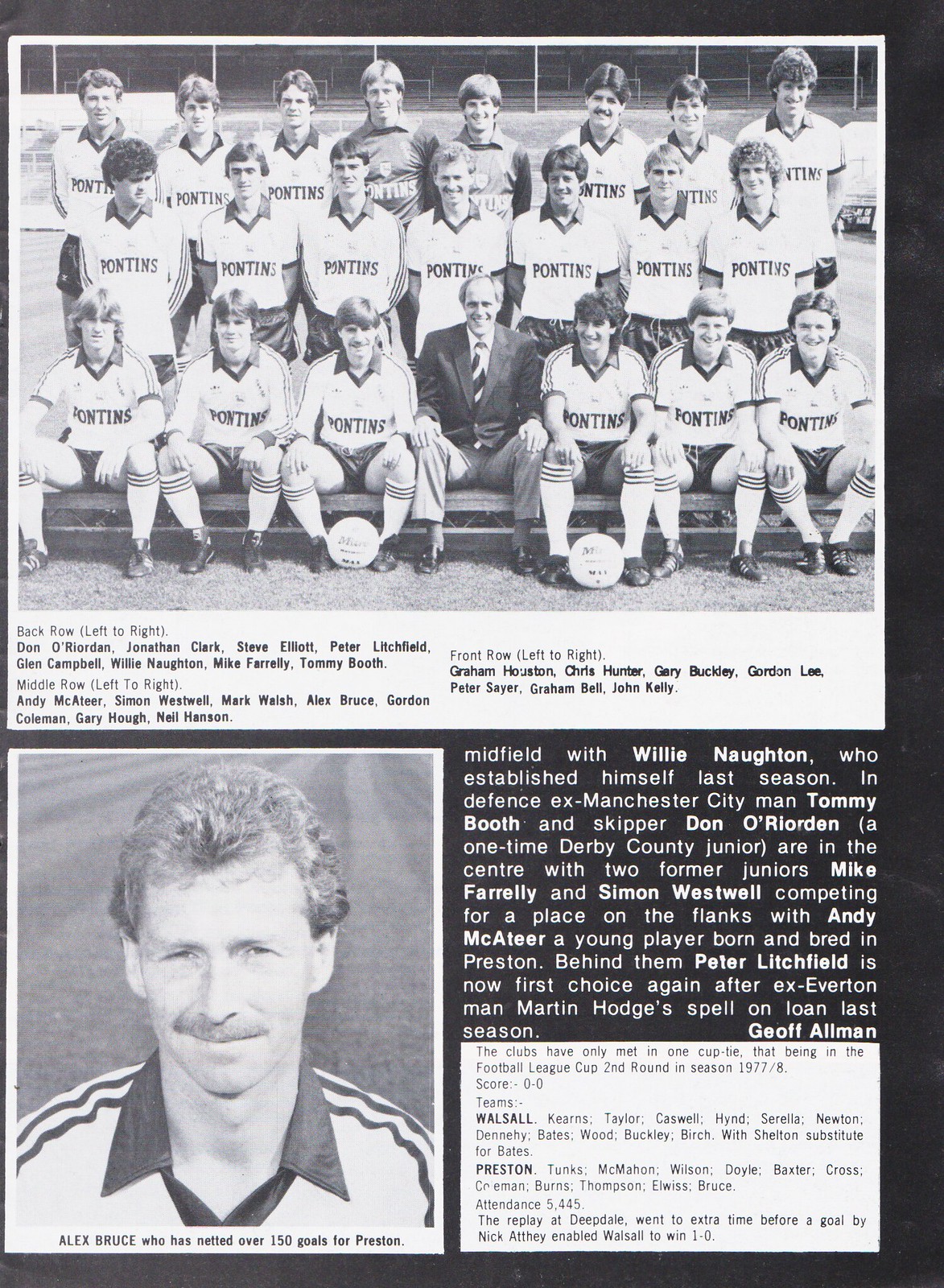The image depicts a black-and-white photo of a soccer team identified as Pontins. The team consists of three rows of players, with the first row seated and the back two rows standing. All players are wearing light-colored kits with colored cuffs on the sleeves and collars. At the center of the front row sits the manager in a suit, flanked by six players and two soccer balls positioned at their feet. Notably, the players include Donna Roden, Jonathan Clark, Steve Elliott, Peter Litchfield, Glenn Campbell, Willie Naughton, Mike Farrelly, Tommy Booth, Andy McEar, Simon Westphal, Mike Walsh, Alex Bruce, Gordon Coleman, Gary Ha, and Neil Hansen. The team lacks diversity, comprising solely white or Caucasian players. Below the team photo, there's a headshot of Alex Bruce, who has netted over 150 goals for Preston, also wearing the same kit. An accompanying article describes key players: Willie Naughton, Tommy Booth, Don O'Riordan, Mike Farrelly, Simon Westwell, Andy McAteer, and Peter Litchfield, with details about their positions and past performances.